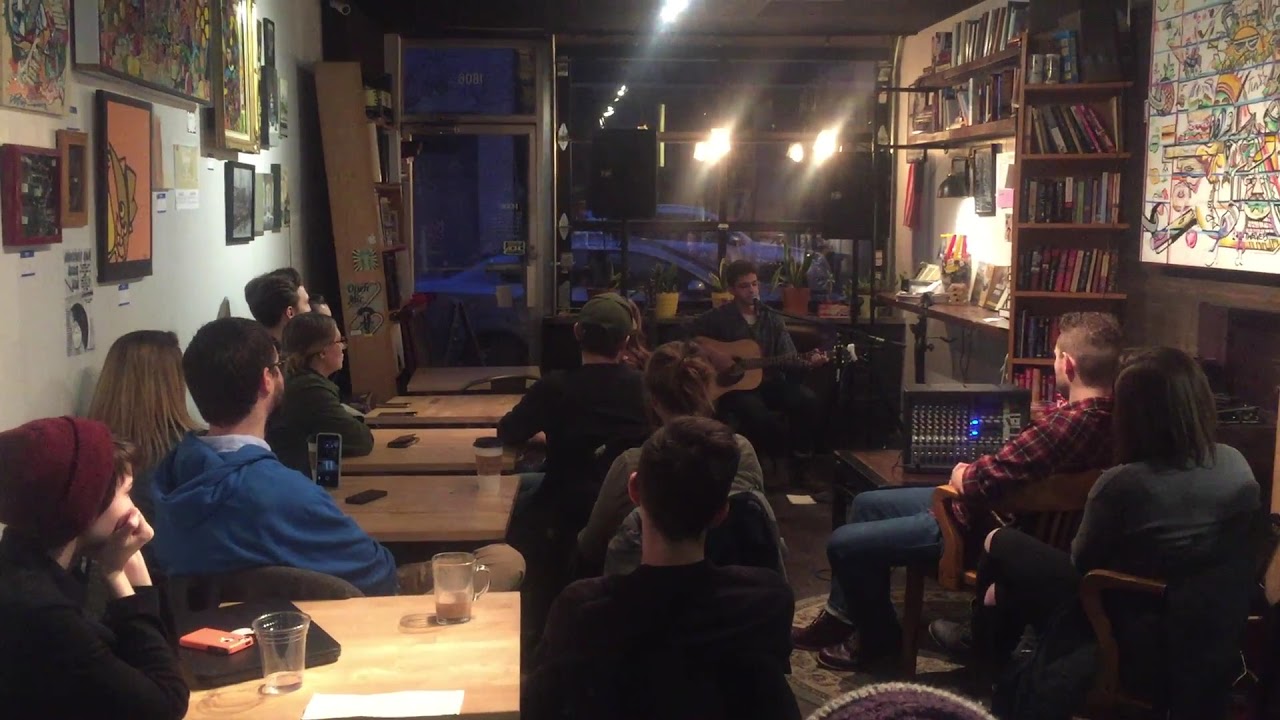In this dimly lit, cozy room that resembles a small cafe or bar, approximately 11-12 people are seated at brown wooden tables, their attention focused on a man in a blue shirt playing a brown guitar. The room features a mix of decor, including a bookshelf on the right-hand wall and a collection of framed pictures and paintings on the left light gray wall. Large glass windows reveal a twilight scene outside, with cars parked on the street and a man with his back to the window, possibly indicating an open door to the street. The atmosphere is intimate, enhanced by spotlights reflecting on the windows and creating a warm ambiance. The crowd, dressed in casual attire including jeans and flannel shirts, seems engrossed in the performance, with glasses on the tables hinting at drinks being enjoyed.